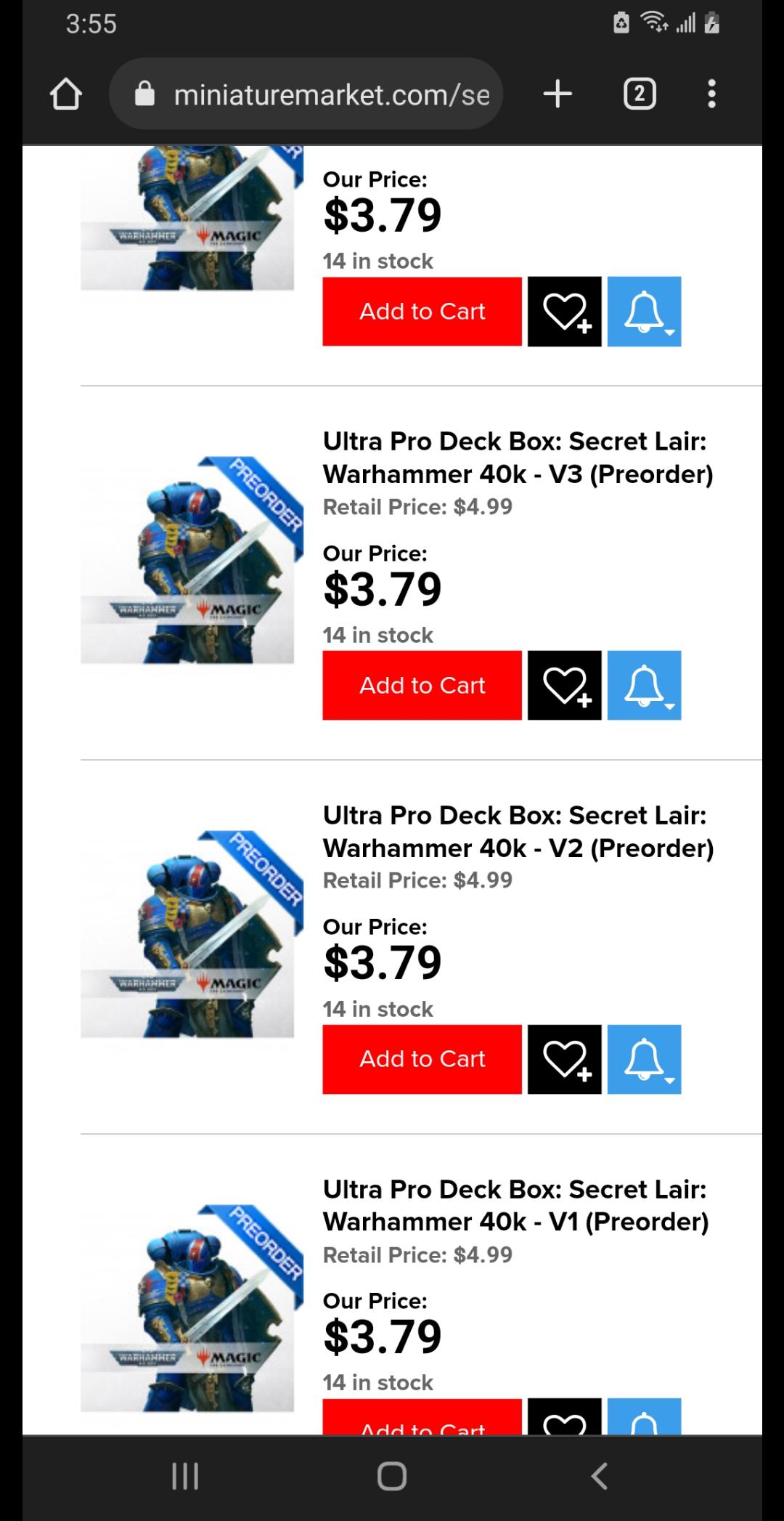The image appears to be a screenshot taken from a cell phone. The background in the far corners, as well as the top and bottom, is black. On the upper left, the time is shown as $3.55. On the upper right, there are five icons, including a battery life indicator. Also on the upper left, there's a house icon next to a lock icon and the partially visible URL of "miniaturemarket.com." Nearby, there is a plus sign, a number 2 inside a box, and three vertical dots, typical for a menu or more options.

Dominating the center of the screen is a large white rectangle, displaying search results for "Ultra Pro Deck Box." Underneath, various listings are shown:
- "Secret Lair, Warhammer 40K, V3" marked as a pre-order with a price of $3.79, indicating there are 14 items in stock.
- Similar listings for "V2" and "V1" are visible as you scroll down.